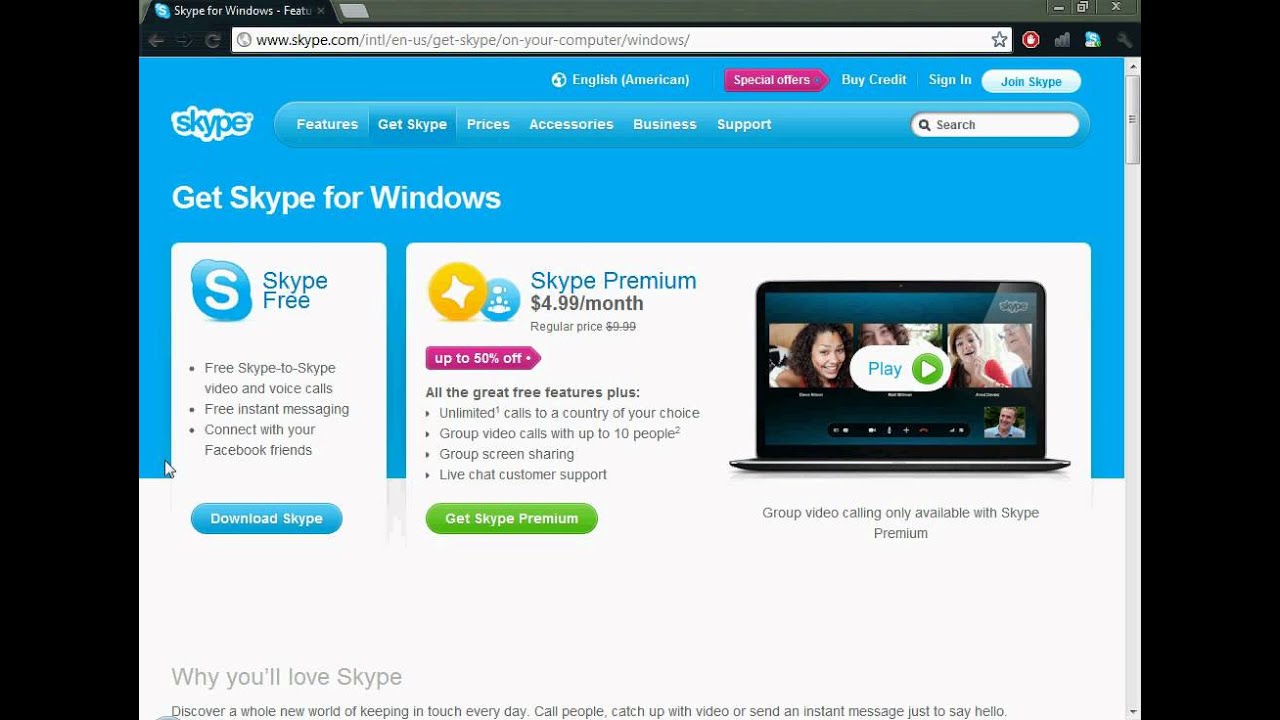The image depicts a web browser with one tab open, displaying the Skype for Windows download page. The URL in the address bar reads "skype.com/intl/en-us/get-skype/on-your-computer/windows". The top two-thirds of the page features a blue banner with the Skype logo prominently displayed. Below the logo, there's a navigation bar with links labeled "Features," "Get Skype," "Prices," "Accessories," "Business Support," and language options, showing "English (American)."

Further down, there are links for "Special Offers," "Buy Credit," "Sign In," and "Join Skype," with "Special Offers" highlighted in red. The rest of the text is white on the blue background, except for "Join Skype," which is written in blue font on a white background.

The highlighted tab is titled "Get Skype," specifically the section for Windows. The blue banner extols the virtues of Skype, such as free Skype-to-Skype video and voice calls, free instant messaging, and the ability to connect with Facebook friends. There is a download button prominently displayed for users to get Skype for their Windows computers.

Below this section, there is an advertisement for Skype Premium, priced at $24.99 per month, marked down from the regular price of $9.99 per month, indicating a 50% discount. The offer includes additional features like unlimited calls to a country of choice and group video calls with up to 10 people.